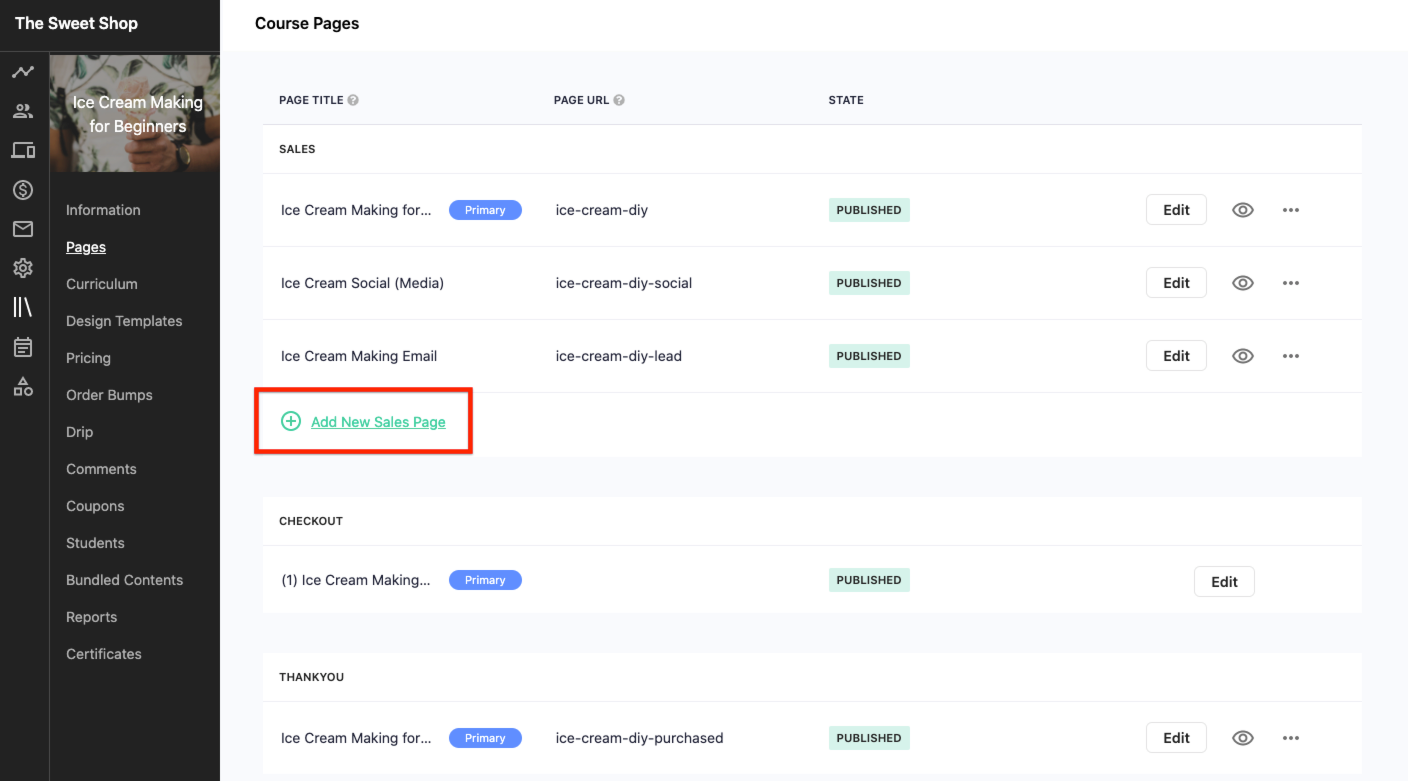This detailed screenshot captures the interface of an online course platform hosting a beginner-level course titled "Ice Cream Making for Beginners." In the upper left-hand corner, the platform is branded as "The Sweet Shop." Directly below the brand name, the course title is prominently displayed, accompanied by a small, likely decorative image.

Beneath the course title, a navigation menu presents an array of options: Information Pages, Curriculum, Design Templates, Pricing, Order Bumps, Drip, Comments, Coupons, Students, Bundled Contents, Reports, and Certificates. These options suggest a comprehensive toolkit for managing and customizing the course content and its delivery.

The central focus of the page is labeled "Course Pages." Below this heading, a table lists essential details about different course-related pages, including the page title, URL, and current state. The highlighted entry, "Sales for Ice Cream Making," has a published state, indicating it's live and accessible to users. Accompanying this entry are menu buttons for further actions, such as editing or previewing the page using the eye icon.

The table contains three similar entries, each with options for editing and viewing. At the bottom of the table, a conspicuous red-highlighted option invites the user to "Add a New Sales Page." Following this, additional options for "Checkout" and "Thank You" pages are available, suggesting the platform supports comprehensive course sales and post-purchase processes. This view likely belongs to the course creator, offering a glimpse into the backend management of the online course.